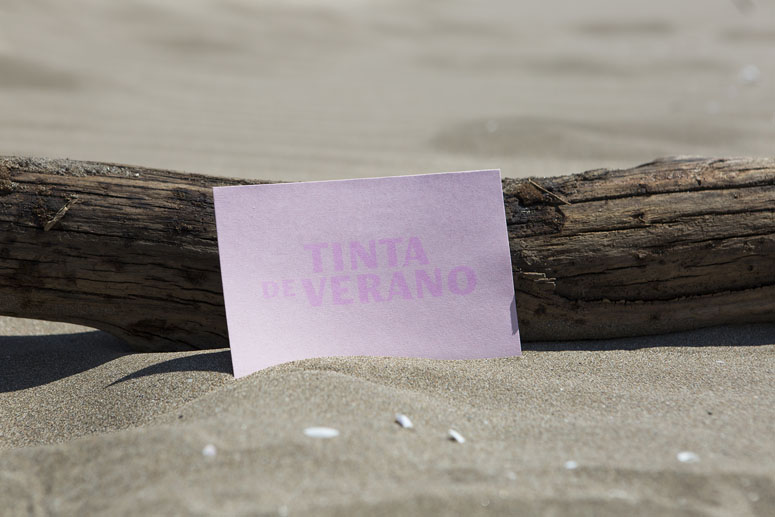The image captures a serene beach setting with finely detailed sandy land encompassing the entire scene. Dominating the middle is an old, weathered brown wooden log placed horizontally, showing distinct horizontal lines and some signs of chipping and rotting. The sand above the log appears out of focus, adding depth to the image, while the foreground sand is perfectly clear, revealing tiny white rocks that enhance the texture. Leaning against this aged log is a white card illuminated by sunlight, casting delicate shadows around it. The card displays the text "Tintor di Verano" in varying shades: the majority of the text is in a light blue or purple hue, with some parts in a brighter pink color, vividly standing out against the white background. The meticulous composition captures the tranquil yet detailed atmosphere of the beach, emphasizing the interplay of light, shadow, and texture.